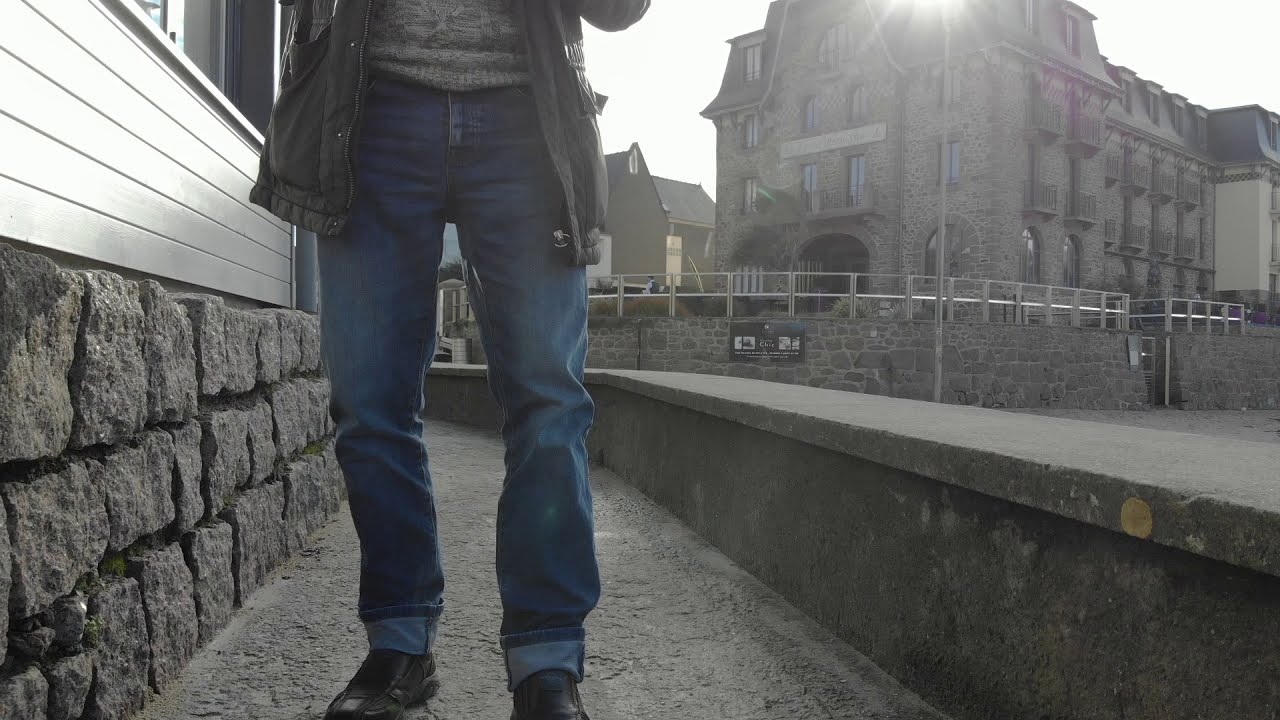In this outdoor photograph, the lower half of a man dominates the foreground, capturing him from the mid-torso down to his feet. He's outfitted in cuffed blue jeans, brown laced shoes, and a fatigue green jacket with pockets that overhangs his hips. Beneath the jacket, he sports a horizontally striped shirt. His arms are raised, as if holding something above the frame. The setting suggests a European urban environment - possibly in London, France, or Belgium - with old-school architecture. 

To the man's left (on the image's right side), a tall, possibly governmental or church-type building looms in the background, with an elevated walkway featuring a steel fenced railing leading up to it. The sky is a solid white, reflecting sunlight at the top of this building. On his right (the left side of the image), there's a house with gray siding sitting atop a gray rock foundation. The ground beneath him appears to be a paved road, bordered by a low cement wall and a section of brick that transitions into the foundation of another building. The scene is devoid of other people, emphasizing the solitary presence of the man against the seemingly timeless urban backdrop.